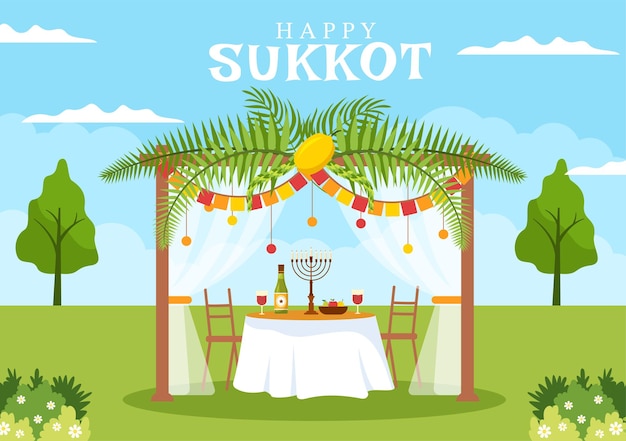The image is a detailed, cartoon-like illustration of a festive Sukkot scene. Two identical trees with dark green trunks and bushy foliage frame the scene on either side. In the background, the sky is bright blue, adorned with white clouds, signifying a sunny day. Below this, a lush, dark pea-colored grass stretches across the image. Under a thatched-roof structure, a picnic table is adorned with a white tablecloth. Central to the table is a Hanukkah menorah, flanked by a wine bottle and two wine glasses, along with a bowl of mixed fruit. Two chairs are positioned at the table. At the bottom corners of the image, there are clusters of bushes with light green, dark green, and cream-colored leaves, accompanied by small white flowers with yellow centers. Above the scene, in bold letters, it reads "Happy Sukkot," marking the Jewish holiday.